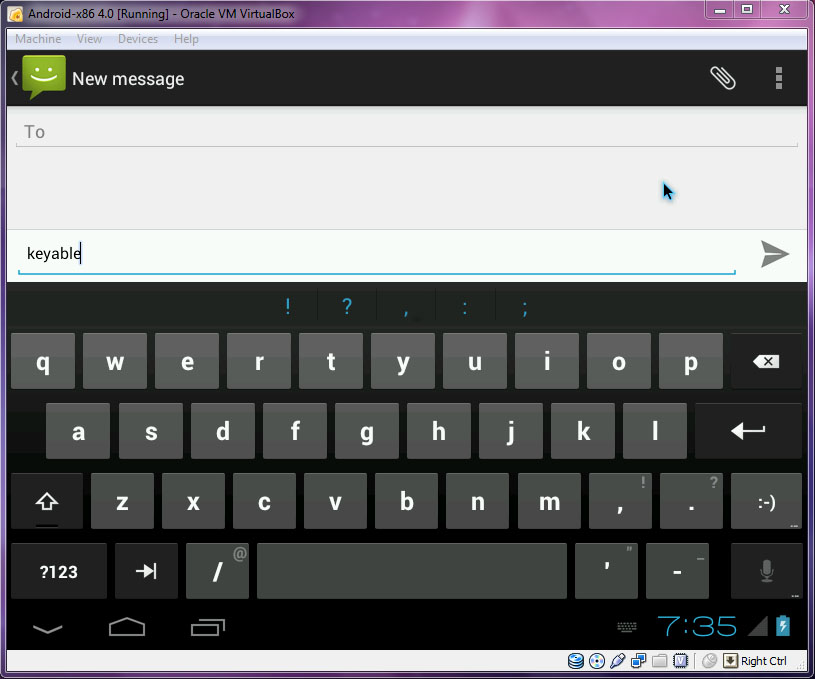The image depicts a screenshot of an Android x86 4.0 virtual machine running within Oracle VM VirtualBox. The Android interface is clearly visible, with a black status bar at the very top displaying typical indicators. Below the status bar is a navigation bar showing that the messaging app is open and in the process of composing a new message. The phrase "new message" appears on the left side of this bar. 

Directly underneath, there's an empty text field labeled "To," where the recipient's contact information is expected to be entered. Following this, a larger text field—intended for the message body—contains the text "keyable." To the right of this field, there is a send icon, which is an arrow pointing to the right, indicating the button used to dispatch the message.

The lower half of the screen is dominated by the virtual QWERTY keyboard. The top row of the keyboard presents special characters and punctuation options, followed by the main QWERTY keys encompassing alphabetic characters across the middle rows. Below these, the space bar spans the bottom with additional keys for switching keyboard modes or symbols situated to its left. Additionally, there is a key featuring a curved arrow, used for return or enter functions.